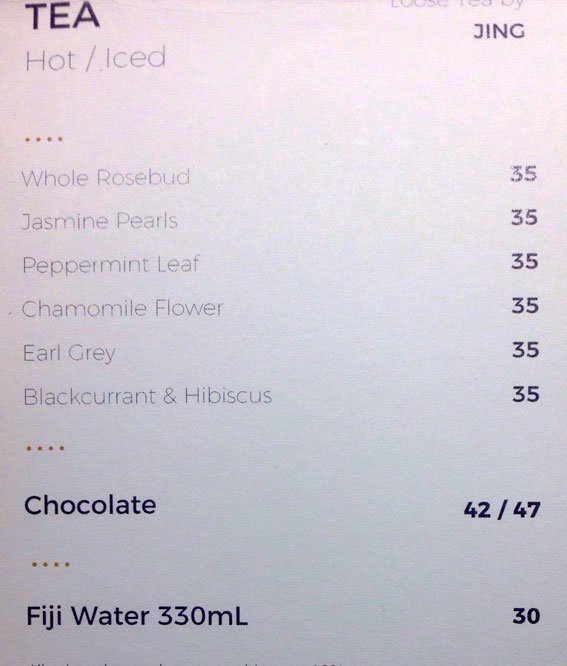The image depicts a clean and simple tea menu set against a white-grayish background. At the top left, the bold title "Tea" is prominently displayed, followed by "hot/iced" in a smaller font directly below it. To the top right, the text "loose tea by Jing" is visible. Moving down along the left side, the first option listed is "whole rosebud," followed by a series of different teas across the menu such as "jasmine pearls," "peppermint leaf," "chamomile flower," "earl grey," and "blackcurrant and hibiscus," each priced at 35. The categories are punctuated with four yellow dots both above and below the section that lists "chocolate," priced at 42/47 depending on the size. At the bottom, another item, "Fiji water 330 milliliters," is listed at a price of 30. The overall design features a minimalist aesthetic with black text and occasional yellow elements to create clear separations between categories.